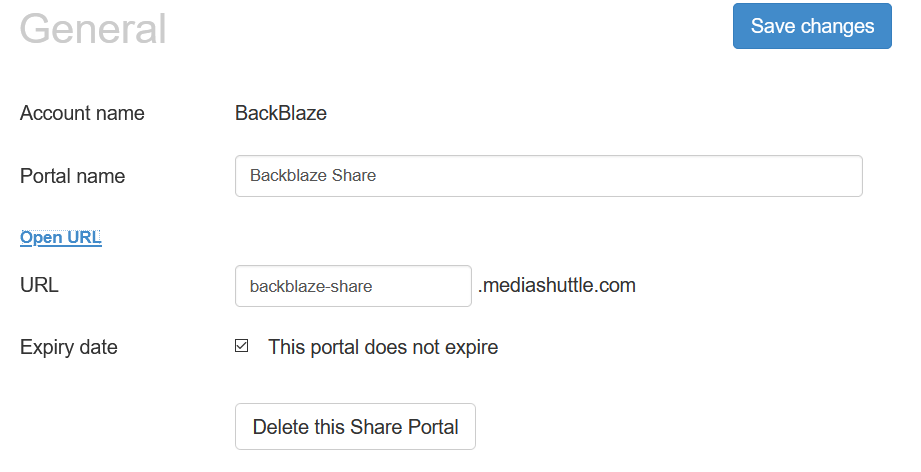The image captures a screenshot taken on a digital device, displaying a settings page with a white background. At the top left corner, in gray print, is the word "General." In the top right corner, there is a blue button labeled "Save Changes" in white text.

Moving down the page, the first section addresses the account name, which is "Backblaze" – written as "Backblaze" with an uppercase "B" followed by lowercase letters, then an uppercase "B" again and lowercase letters. The next section addresses the portal name, labeled "Backblaze Share."

Beneath the portal name section, an option labeled "Open URL" appears on the left side, underlined in blue, indicating a clickable link. To the right is a box containing the URL "backblaze-share.mediashuttle.com."

Further down, there is a section for the portal's expiry date, stating, "This portal does not expire," with a checkmark in a box next to it.

At the bottom of the page, there is a clickable black-printed box labeled "Delete this Share Portal."